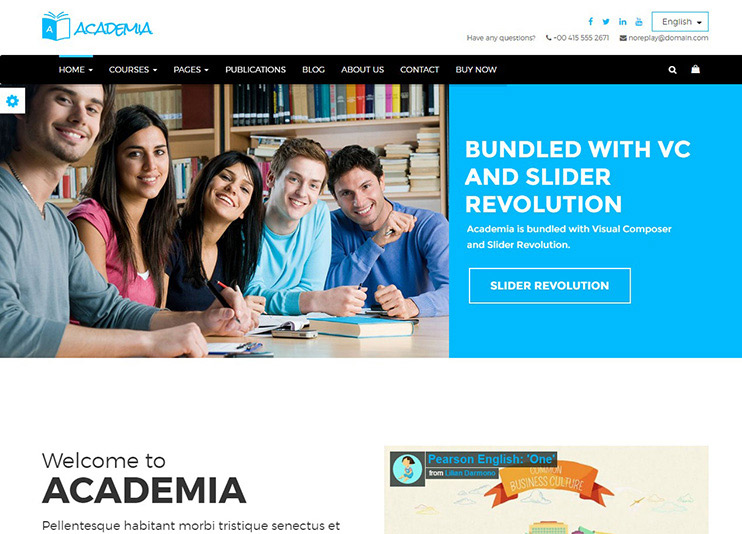This is a detailed description of the visual elements depicted in the image of a website:

The image showcases the homepage of a website named "Academia". The website's title "Academia" is prominently displayed in the top left corner in blue. Adjacent to it on the right are icons for social media platforms: Facebook, Twitter, and LinkedIn. Further right, there is a language selection option, currently outlined around "English".

Below these elements are three call-to-action options: "Have any questions?" followed by a question mark, a phone number, and an email address listed as **nodisplay@domain.com**.

The background around the navigation categories is black. The navigation menu runs horizontally from left to right and includes the following categories: Home, Courses, Pages, Publications, Blog, About Us, Contact, and Buy Now. To the right of these categories, there is a search bar accompanied by a shopping bag icon.

Central to the image is a photograph of five smiling people posing for the camera, with a bookshelf in the background. The group comprises three males and two females.

To the right of the photograph is a light blue square with text indicating "Bundled with VC and Slider Revolution" in white. Below this, there is text confirming that "Academia is bundled with Visual Composer and Slider Revolution". Further down, a rectangular outline in white contains the text "Slider Revolution".

The rest of the background is predominantly white. There is a large welcome message that says "Welcome to Academia," followed by a series of words and acronyms: Plentesk, Pabot, Morby, Triskew, Synectis, EC - which are not in English. To the right of this text is the word "Pierce" in English, followed by "1" with a label resembling a gold ribbon against a lighter gray background.

This comprehensive summary captures all the details visible on the website screen displayed in the image.